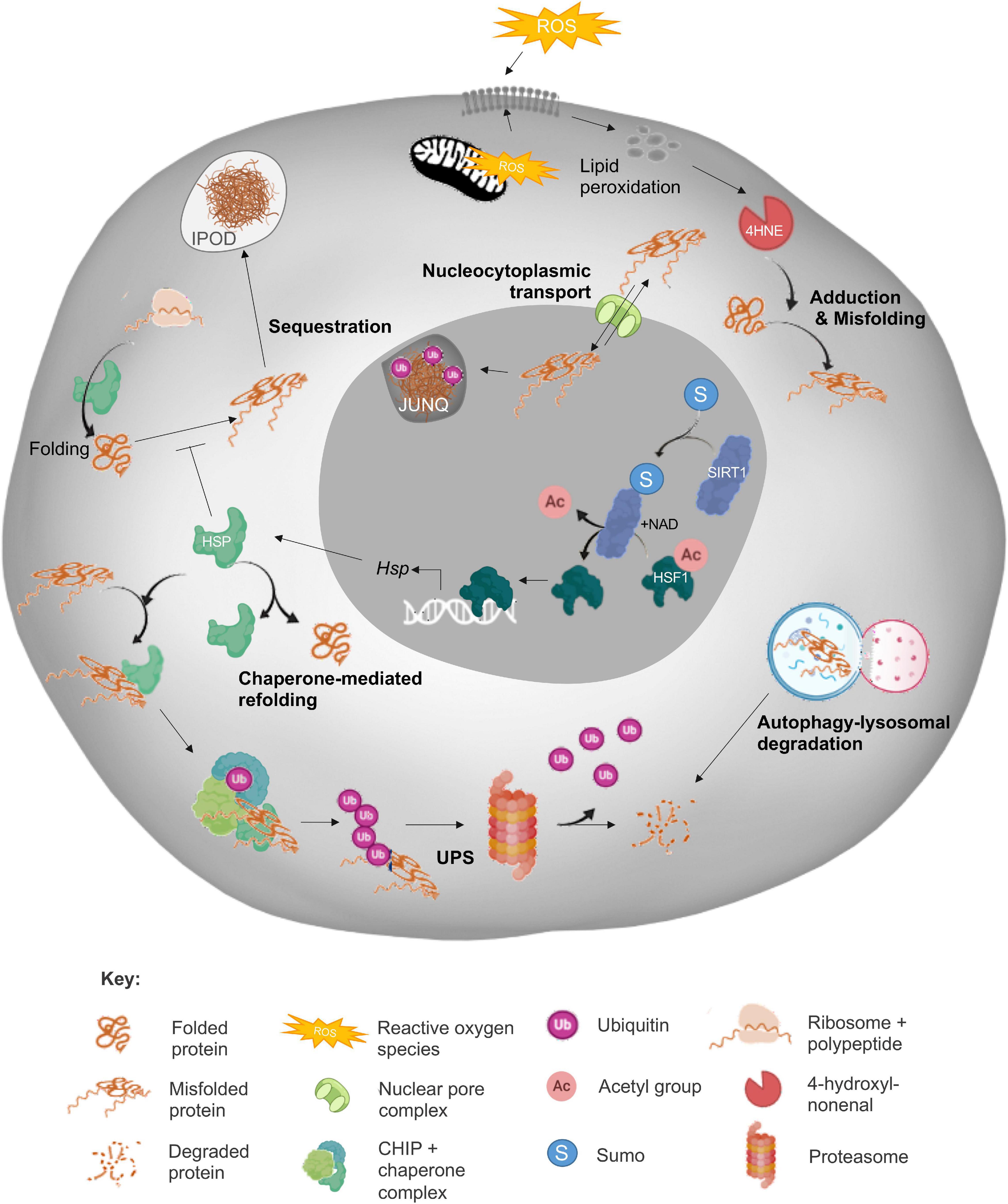This infographic presents a detailed diagram related to biological processes, primarily focusing on protein dynamics and cellular interactions. The visual consists of two concentric gray circles, with the inner circle being darker gray and the outer circle lighter gray. 

Inside the lighter gray circle, starting from the bottom right and moving counterclockwise, are labels such as "autophagy, lysosomal degradation," followed by arrows pointing towards "UPS," and continuing to terms like "chaperone mediated refolding," "sequestration," "nucleocytoplasmic transport," "liquid peroxidation," "adduction," and "misfolding." The darker gray circle contains multiple 'S' symbols in blue, pointing towards a distinct image labeled "AC," which then points to "HSP." The upper part of the circle features "JUNQ."

The diagram includes numerous small illustrations depicting various cellular components and protein states. These include a brown coiling string labeled "folded protein," a yellow explosion graphic marked "reactive oxygen species (ROS)," a purple circle with "UB" representing "ubiquitin," a wavy brown line in a pink sandwich indicating "ribosome plus polypeptide," a jagged brown string as "misfolded protein," and a green semi-circle for "nuclear pore complex." Additional symbols include a pink circle with "AC" for "acetyl group," a pie chart-like figure labeled "4-hydroxy-2-nonenal," a fragmented string tagged "degraded protein," a green figure surrounded by blue bits named "CHIP plus chaperone complex," a blue circle with an 'S' for "SUMO," and a coiled rope-like figure for "proteasome."

At the bottom, a key explains these images in detail, aiding in understanding the complex interactions shown by the diagram. The diagram visually connects these elements with arrows and labels to demonstrate processes such as sequestration, adduction, misfolding, and others, providing a comprehensive overview of protein lifecycle and cellular maintenance mechanisms.